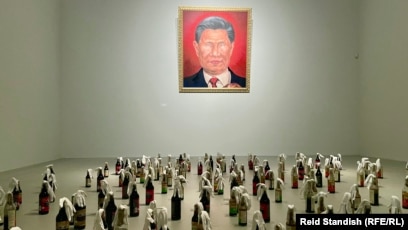The image depicts a large, eerily empty room with pale, greyish-white walls that tower approximately 30 feet high, emphasizing the vast, minimalistic space. Dominating the scene is a large photograph of a man with short black hair, a black jacket, white shirt, and red tie, set against a vivid red background. The photograph is enclosed in a gold frame and mounted high on the wall. At the bottom of the photograph, the text reads "Red Standish." 

In the center of the room stands a crowd of about 100 people, all wearing long white gowns and veils reminiscent of Arabic customary clothing, adding to the haunting and surreal atmosphere. The people, dressed in these uniform garments, stand in stark contrast to the otherwise bare room and the single, imposing portrait.